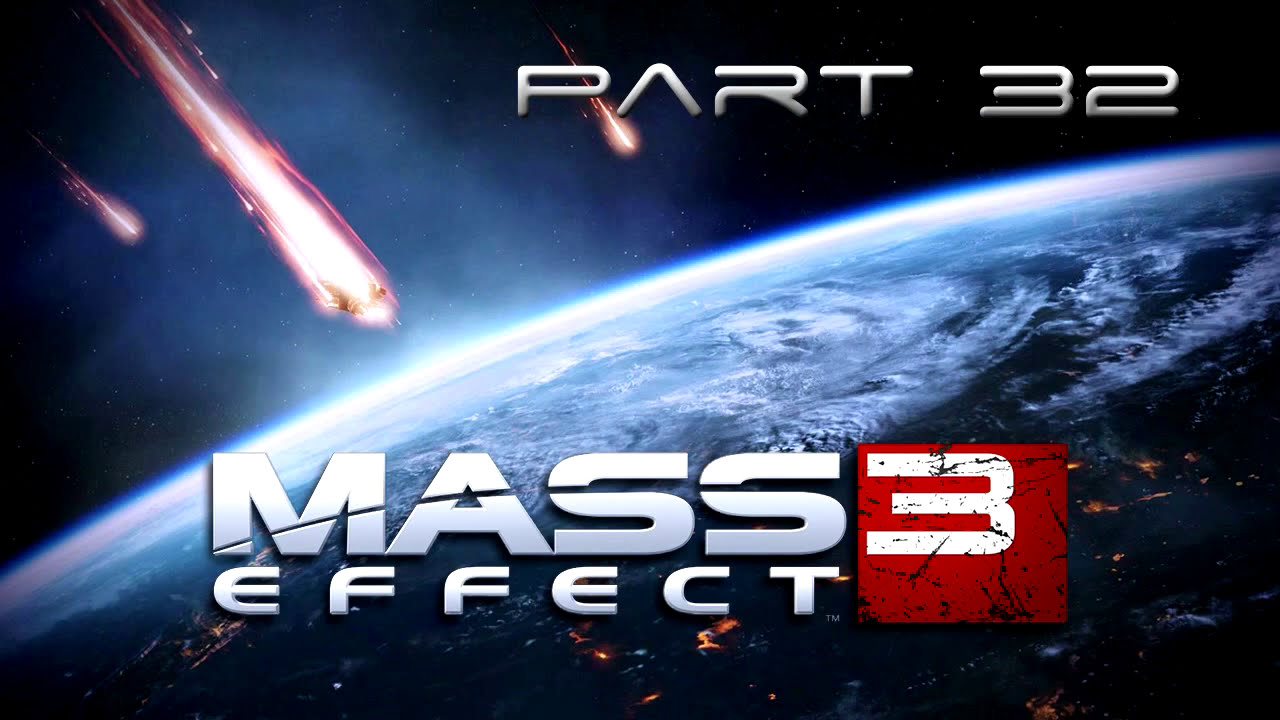This image serves as a detailed, sci-fi-themed YouTube thumbnail for the video game Mass Effect 3, specifically marking "Part 32" of what appears to be a video series or livestream session. Dominating the frame is a striking, blue Earth-like planet, depicted against the stark blackness of space. The planet's surface is layered with white clouds and enveloped by a thin, blue atmospheric haze. Dramatically approaching the atmosphere are three to four large fiery meteors, seemingly on a collision course. The iconic "Mass Effect 3" logo is prominently displayed at the bottom of the image. The text "Mass Effect" appears in sleek, modern, silver letters, while the number "3" is highlighted within a distinct red square. The lettering style and colors embody the futuristic and intense theme of the game. The "Part 32" label in the top right corner, written in a stylistic, possibly alien-like font, further emphasizes the episodic nature of the content.